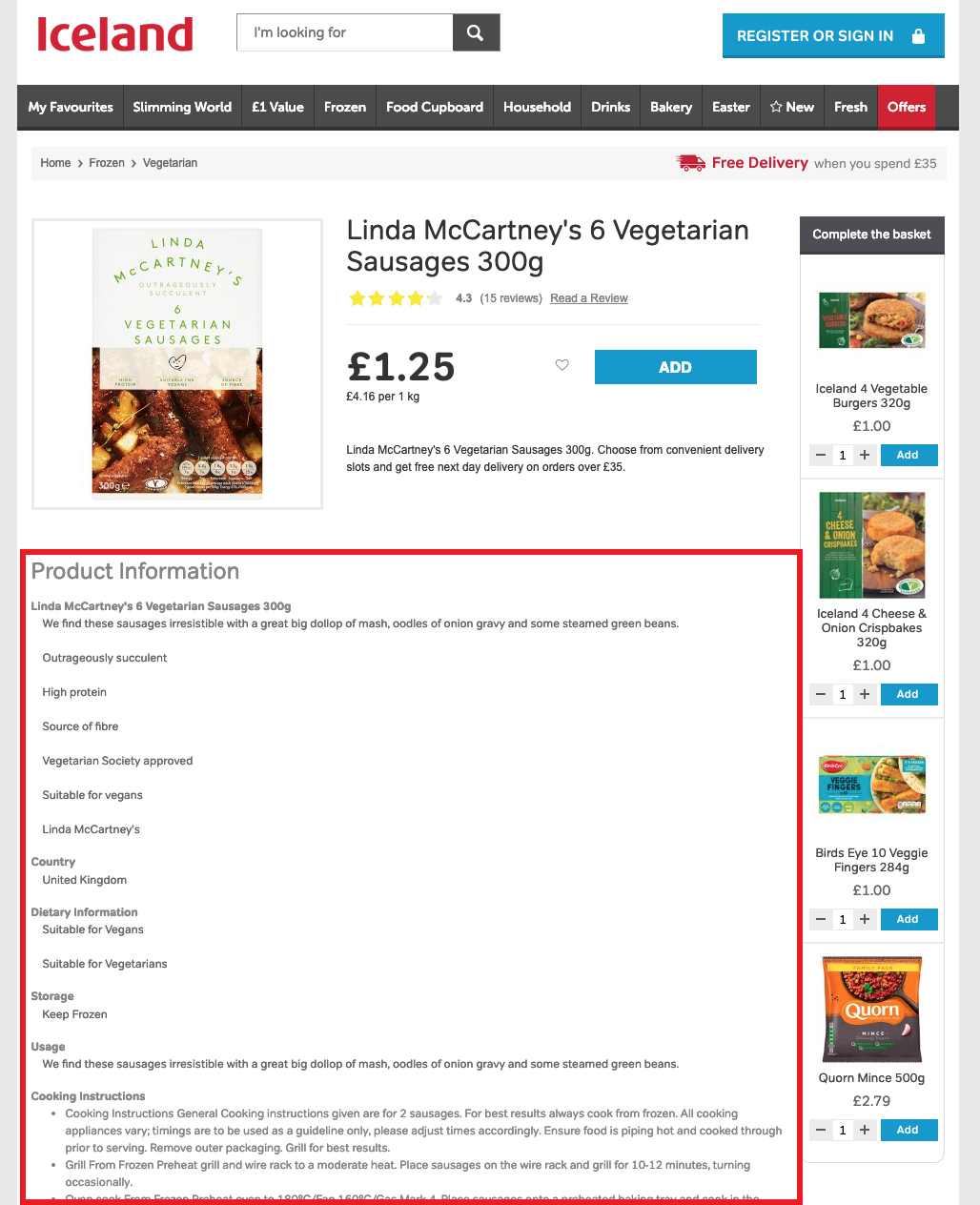Here is an improved and detailed version of the caption:

---

This image features a website interface dedicated to an online grocery store. In the upper left-hand corner on a white background, the logo "Iceland" is displayed in bold red text. Adjacent to the logo is a search box, and on the far right side, there is a blue button labeled "Register or Sign In". 

Directly below, a gray-bordered navigation bar offers several clickable options including "My Favorites," "Slimming World," "One Euro Value," "Frozen," "Food Cupboard," "Household," "Drinks," "Bakery," "Easter," "New," "Fresh," and "Offers."

Underneath the navigation bar, a section titled "Home" features the "Frozen" category. Highlighted is the product "Linda McCartney's 6 Vegetarian Sausages, 300g" priced at £1.25. Beside this is a blue "Add" button. The accompanying text promotes the product as "Linda McCartney's 6 Vegetarian Sausages". It also mentions convenient delivery options, including free next-day delivery on orders exceeding 35 pounds or euros.

A red banner provides detailed product information. The description reads, "Product information: Linda McCartney's 6 Vegetarian Sausages, 300g. We find these sausages irresistible with a great big dollop of mash, oodles of onion gravy, and steamed green beans. Outrageously succulent, high protein, source of fiber, Vegetarian Society approved, suitable for vegans."

Further details include:
- Manufacturer: Linda McCartney's, United Kingdom
- Dietary Information: Suitable for vegans and vegetarians
- Storage Instructions: Keep frozen
- Usage: "We find these sausages irresistible with a great dollop of mash, oodles of onion gravy, and steamed green beans."
- Cooking Instructions: Provided for two sausages, with general guidelines to cook from frozen for the best results. Variations in cooking appliances might require adjustments in cooking times. Ensure food is piping hot and cooked through before serving. Recommended to remove outer packaging and grill for optimal results.

---